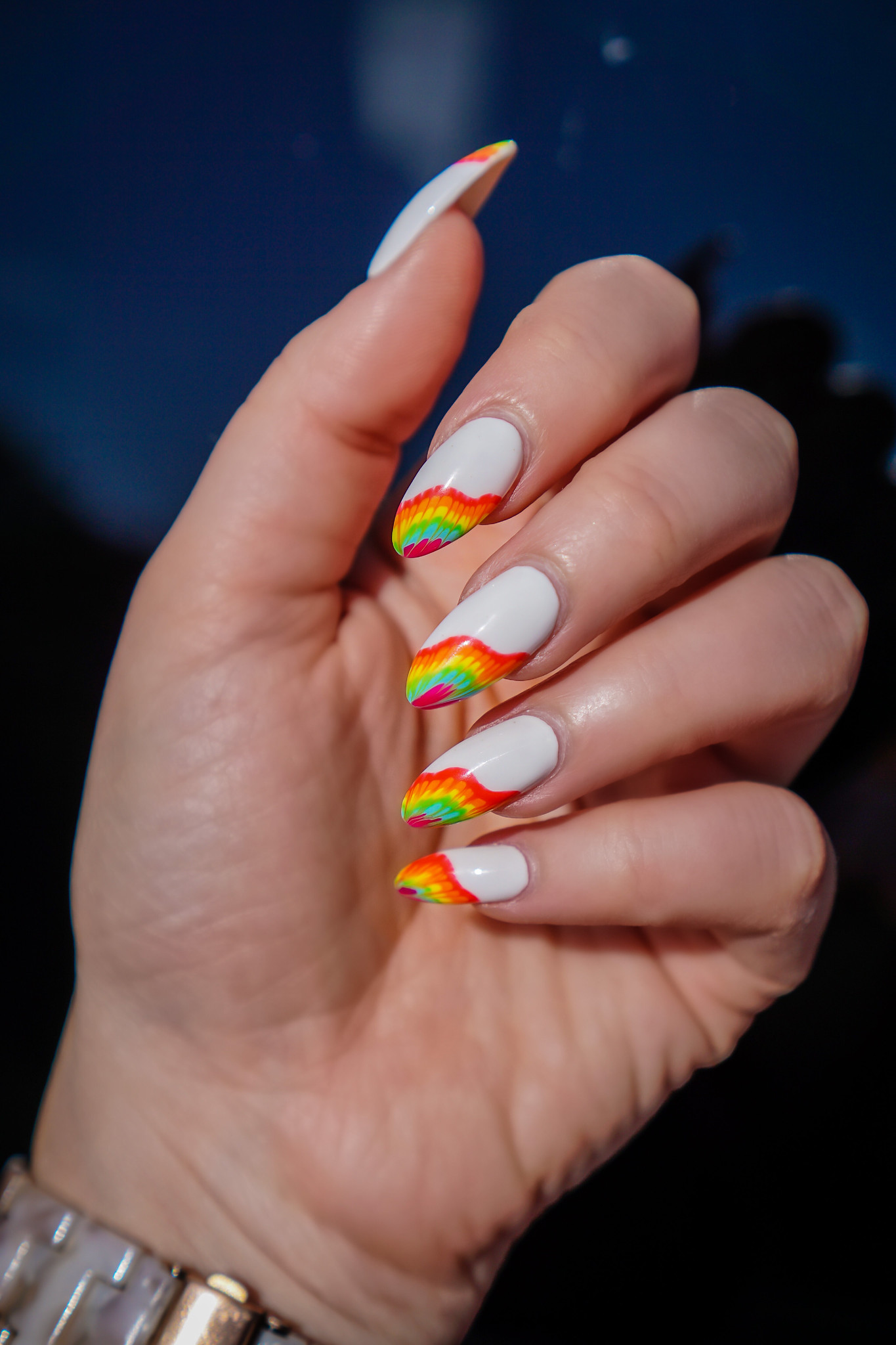A close-up image showcases a centrally placed Caucasian hand with all fingers visible, featuring freshly done nails. The nails, painted white, have colorful tips that transition from red, orange, yellow, green, blue, to pink, running from the middle to the edges. The person wears a gold and silver metallic wristwatch. The hand casts a shadow onto its palm, emphasizing the illumination in the setting. The background is a night sky, blue in hue, with dark shadows occupying the lower part. A white glowing object is visible at the top of the image, enhancing the overall ambiance.